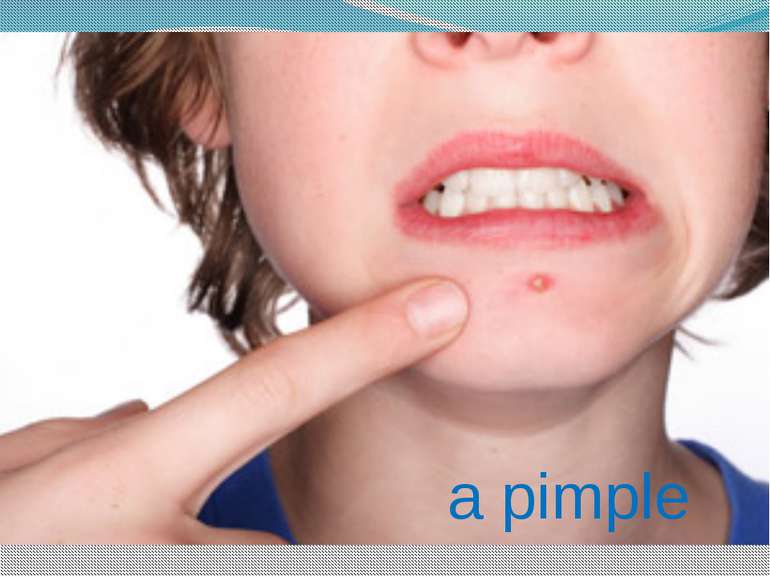The photograph depicts a young, white-skinned teenager from the nostrils down to the top of their shoulders, set against a pure white background. The teenager, whose wavy, chin-length brown hair suggests a bob style, has their mouth slightly open with clenched teeth visibly pressed together, revealing the upper and lower rows of white teeth. Wearing a blue shirt, they are using their right hand to point towards a prominent pimple located between their lower lip and chin. The pimple is notably red with a whitehead, indicating it's about to burst. The teenager's face expresses concern or discomfort about the blemish. Their short fingernails, particularly on the pointing index finger, are visible. In the bottom right corner of the image, on top of the neck area, blue lowercase text reads "a pimple." The overall image has additional design elements: a light blue strip with black dots at the top, and a white strip with black dots at the bottom.